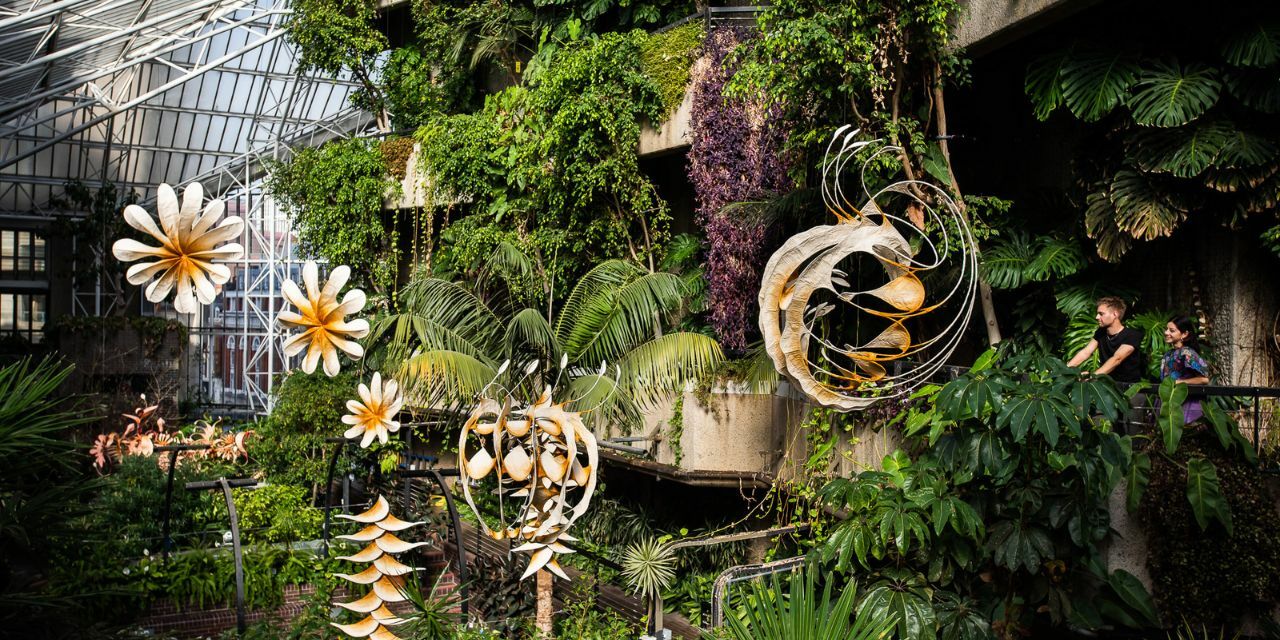The photograph captures a lush, expansive botanical garden housed within a massive glass enclosure. The left side of the image reveals both the steel structure and glass roof of the building, providing a sense of the immense space. On the right-hand side, two people—likely a man and a woman—are seen leaning over a rail, appearing small against the backdrop of towering tropical foliage. Their gaze is fixed on a verdant jungle of various plants and multi-shaped, abstract decorations interwoven among the greenery.

Dominating the scene are tropical trees, including a prominent palm, and large leaves, likely from fan plants. Hanging amongst these are several eye-catching pieces of art, possibly mistaken for real flowers. The flowers in question are large, predominantly white with orange centers, and although striking, they appear to be part of the artistic display rather than genuine flora. Additional decorations with curly, odd, and roundish shapes add to the surreal atmosphere of this indoor paradise.

In the distance, a silver fence subtly peeks through the dense forest of foliage, contributing to the sense of an enclosed yet vast and immersive environment. Vines hang from what looks to be a three to four-story structure, reinforcing the sheer scale of this botanical wonderland.